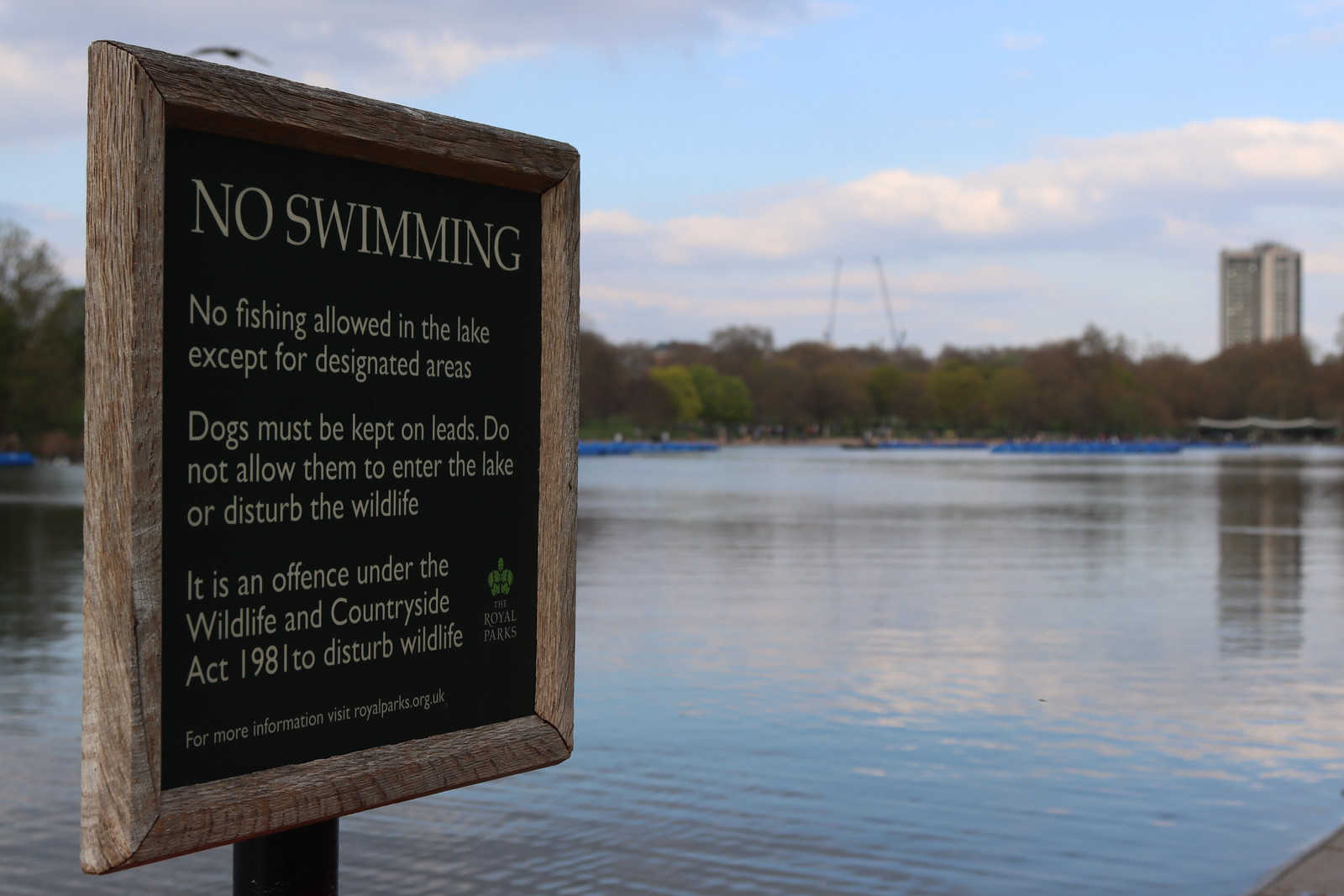The image depicts a serene lake set against a backdrop of dense trees at the far end, under a bright blue sky partially covered with white and gray clouds. The location is captured from the lake shore, presenting a panoramic view of the entire scene. To the right, in the distance, a skyscraper peeks above the treeline, contributing an urban element to the otherwise natural landscape. 

In the immediate foreground, a wooden-framed sign stands posted on the edge of a pier. The sign, detailed with a green logo of "The Royal Parks," prominently conveys important rules: "No swimming," "No fishing allowed in the lake except for designated areas," and "Dogs must be kept on leads." It also warns against disturbing the wildlife, citing the Wildlife and Countryside Act 1981, with information directed to royalparks.org.uk.

The surface of the lake shimmers as sunlight dances across the water, adding a touch of radiance to the tranquil environment. Hidden within the distance of the photo, a few long blue rowing boats skim the surface of the water, blending seamlessly with the natural and urban surroundings.